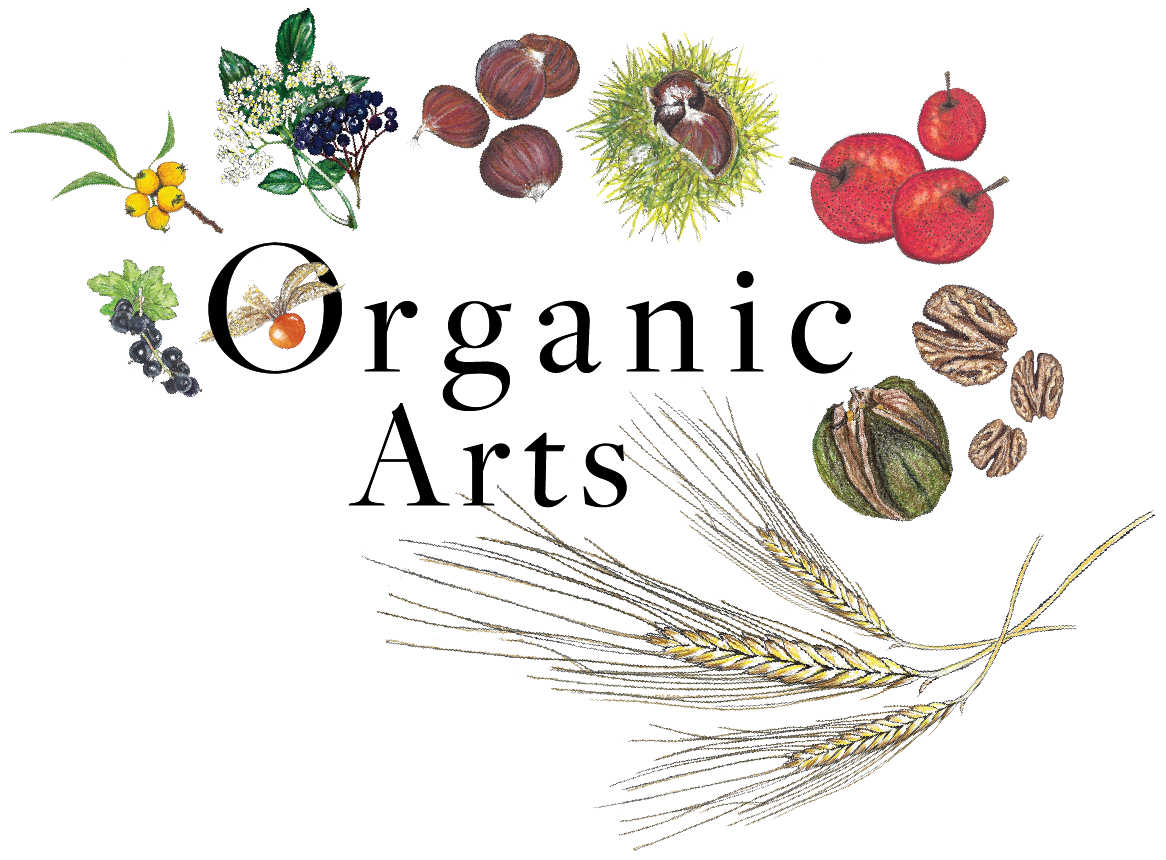This illustration, possibly created with pen and watercolor, features a detailed and vibrant arrangement of various fruits, nuts, and vegetables against a white background. Central to the image is the black serif text "Organic Arts," with "Organic" on the top line and "Arts" underneath, both using capitalized 'O' and 'A'. Surrounding this text are meticulously drawn organic items arranged in a circular pattern.

On the left side, there are clusters of blueberries and yellow gooseberries, while towards the center are some white flowers interspersed with blueberry-like dots. Also present are illustrations of chestnuts or water chestnuts, both whole and encased in green shells.

The bottom right features three lightly colored yellow wheat stalks. Above these are a walnut within its green husk and three more shelled walnuts. Red tomatoes or cherries are depicted above the walnuts. To the top, there are green grassy elements with brown centers and clusters of brown nuts resembling acorns. Further left, a green plant displays white flowers and more blueberries. Adjacent to this are green leaves and yellow lemons or gooseberries.

Besides these, inside the 'O' in "Organic" is a small red berry, connected to a white branch. To its left, a green leaf with bunches of small black berries extends from the margin. Thin graphic lines outline all these ingredients, adding a detailed touch to the entire composition. The illustration combines a mix of colorful organic produce, creating a harmonious and intricate portrayal of natural foods.